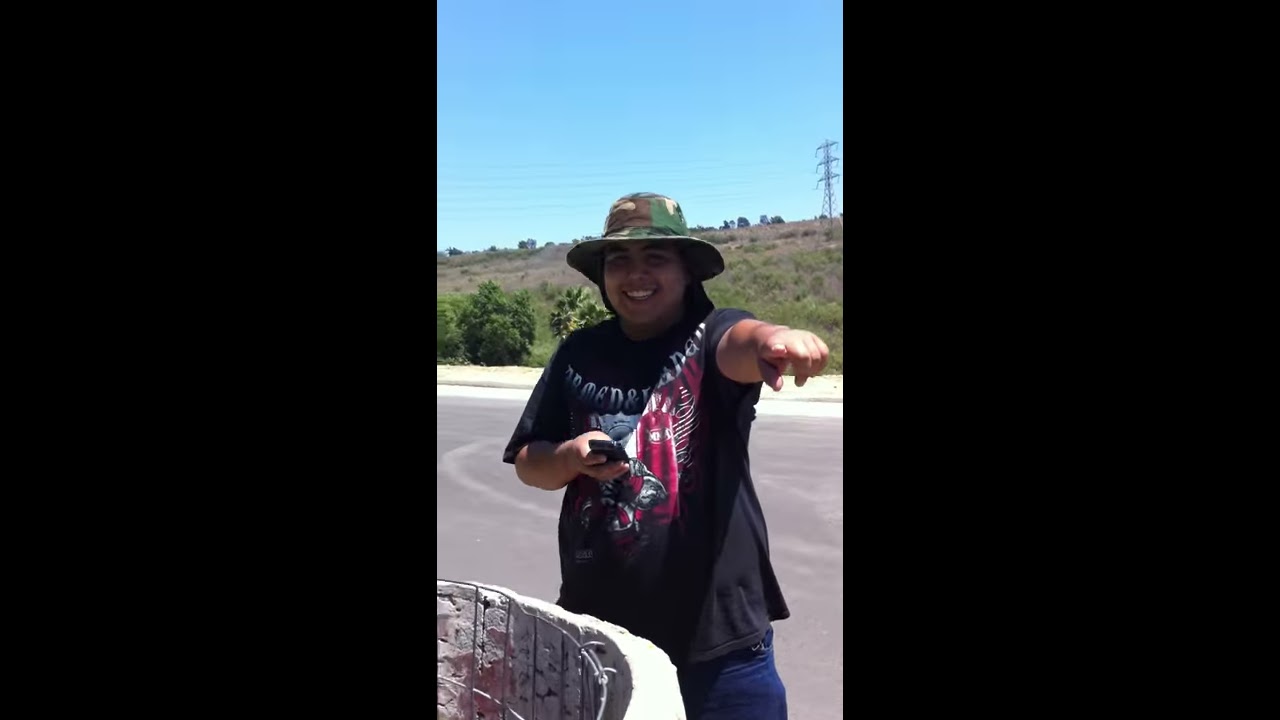This outdoor image captures a smiling, dark-haired woman pointing towards the camera. She stands at the center of the image, dressed in a camouflage sun hat, a black t-shirt with white lettering and red designs that are not fully legible, and dark blue jeans. Her left arm extends towards the viewer in a pointing gesture, while her right arm is bent at the elbow, holding a cell phone. In the lower left corner of the image, there is a small, round concrete structure with a metal wiring insert. Directly behind her is a gray roadway, with visible tracks suggesting vehicle usage. Beyond the road, a hill rises in the background, covered with both green shrubs and patches of dying brown grass. To the top right, an electrical power line tower stands tall against a light blue sky. The scene appears to be a casually taken photograph, highlighting a simple, everyday outdoor setting.